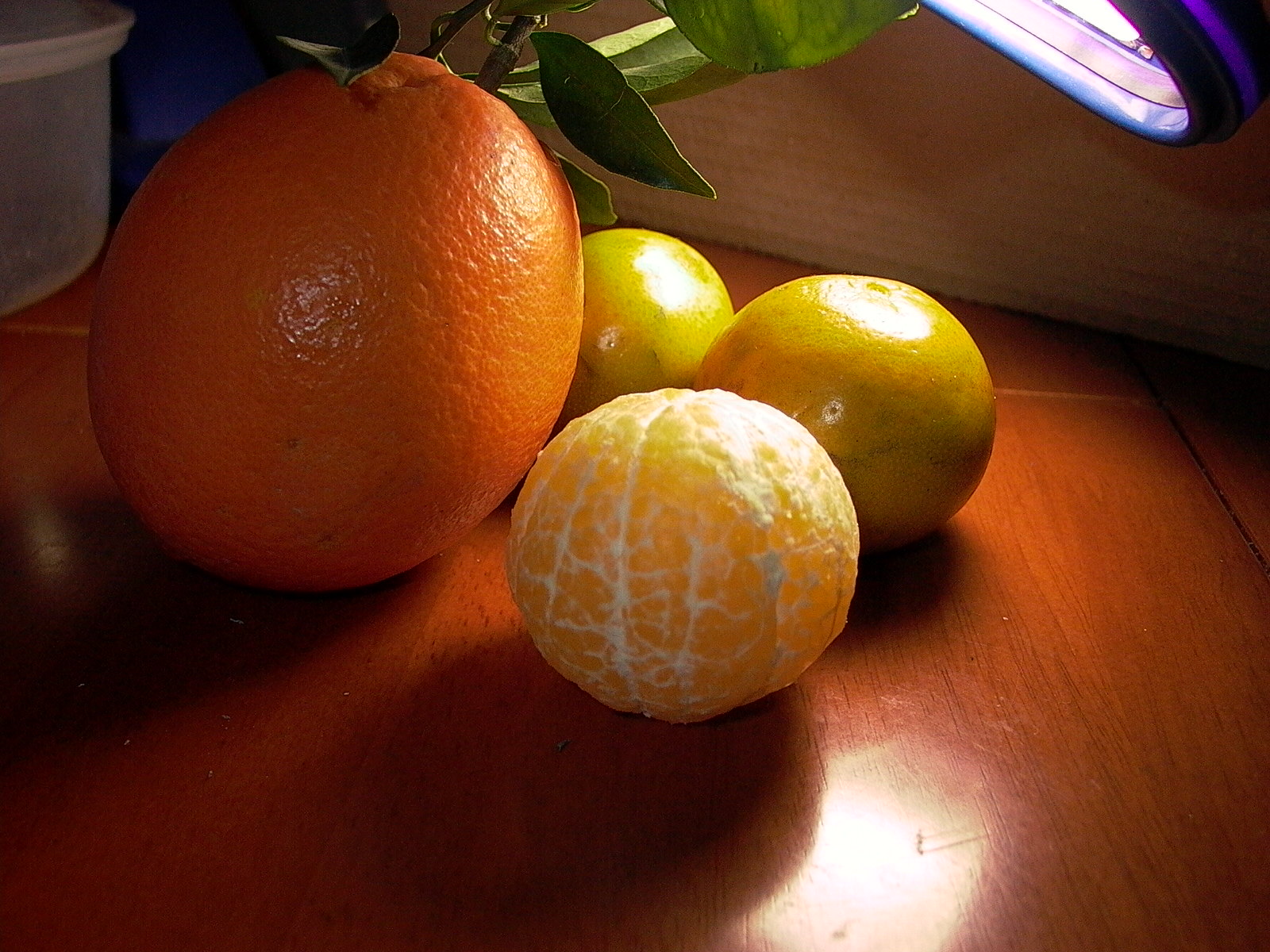In the center of this indoor photograph, a striking array of fruits is meticulously arranged on a brown, cherry wood laminated table. Starting on the left, a large navel orange with a bumpy texture and a couple of green leaves at the top sits prominently. Directly next to this orange is an unpeeled mandarin orange, revealing its white fleshy, pulpy areas. Behind the unpeeled mandarin, two shiny green apples catch the viewer's eye. These items are illuminated by a circular fluorescent desk lamp positioned in the upper right corner, casting a clear, focused light that enhances the vibrant colors of the fruits. The background features what appears to be a wall that resembles corrugated cardboard, adding an interesting texture to the scene. Additionally, a green plant with lush leaves can be seen partially behind the fruits, contributing a touch of nature to this artistic composition. The entire setup is meticulously lit, emphasizing each fruit's distinct characteristics and creating a visually appealing harmony.